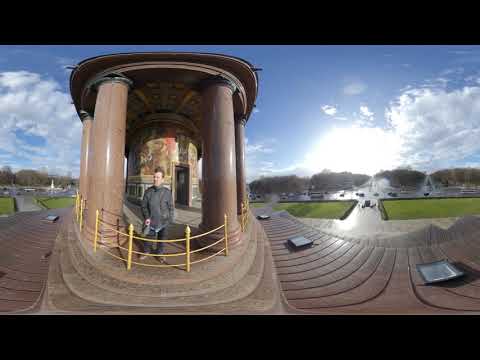In the image, a male wearing a gray jacket and gray pants with sneakers is standing at a large monumental structure that features light beige pillars. He is positioned between two of these pillars and in front of a small yellow metal fence, with stairs leading up to the monument. The monument, resembling a Parthenon or a mausoleum, is centrally located in the frame. A pinkish sidewalk leads up to the structure on the right side. The surroundings include a vast wooden deck at the bottom, a distant grassy area with trees, a large parking lot on either side of the monument, and buildings and cars further in the distance. The sky is bright blue with fluffy white clouds, indicating a clear daytime setting, possibly late evening as the sun is low. The image is taken with a fisheye lens, adding a dramatic, curved distortion to the scene, which enhances the perception of depth and curvature of the structure. There is no text within the image. The colors present include black, blue, white, gray, brown, tan, orange, and yellow.